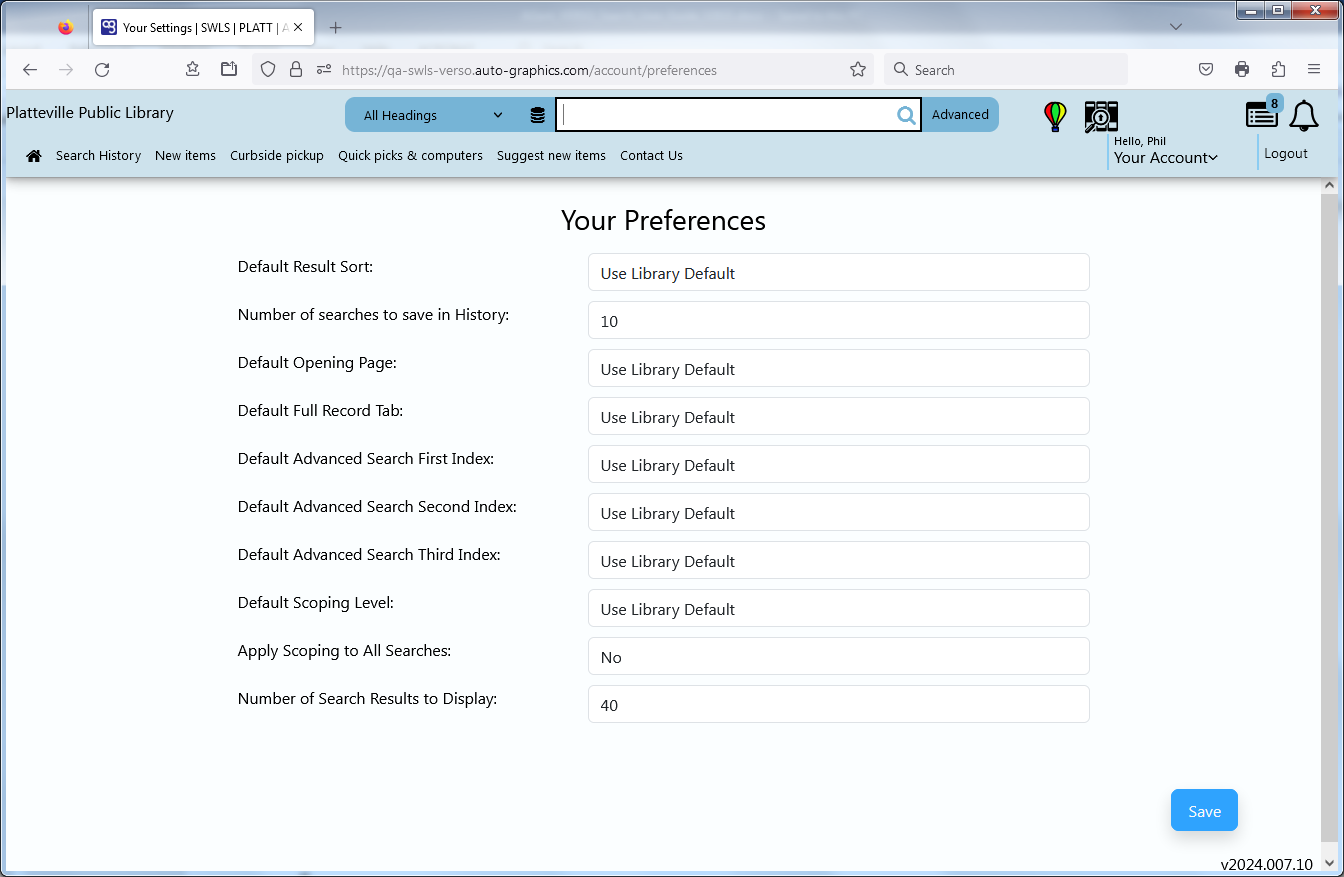**Caption:**

This screen capture showcases the account preferences page of a website with the URL [https://qa-swls.dash.versoautographics.com/account/preferences](https://qa-swls.dash.versoautographics.com/account/preferences). The browser window displays several standard icons including arrows, a refresh icon, a star, a shield, a paddle, a search box, an envelope, and a printer icon.

Dominating the upper section of the webpage, in a light blue box with black font, the header reads "Platteville Public Library." Below this, the navigation menu includes options such as "Search History" (featuring a house icon), "New Items," "Curbside Pickup," "Quick Picks and Computers," "Suggest New Items," and "Contact Us." Above this header, a darker blue box houses a set of dropdown menus with choices including "All Headings," next to a white search box, a blue magnifying glass icon, and a blue box labeled "Advanced." Additionally, there's a multicolored hot air balloon icon and what appears to be a filmstrip with a magnifying glass icon.

User-specific options are present with the greeting "Hello, Phil," accompanied by a dropdown menu labeled "Your Account" and a newspaper-like icon displaying the number eight in blue and black. Following this is a black outlined bell icon.

In the main content area, the background is white with black font text dedicated to various user settings. Each setting features a dropdown menu on the right side. The settings listed include:

- **Default Results Sort:** Uses library default
- **Number of Searches to Save in History:** 10
- **Default Opening Page:** Uses library default
- **Default Full Record Tab:** Uses library default
- **Default Advanced Search First Index:** Uses library default
- **Default Advanced Search Second Index:** Uses library default
- **Default Advanced Search Third Index:** Uses library default
- **Default Shopping Level:** Uses library default
- **Apply Scoping to All Searches:** No
- **Number of Search Results to Display:** 40

These options are followed by a blue "Save" button with white font. At the bottom of the page, the version number is indicated: v2024.007.10.